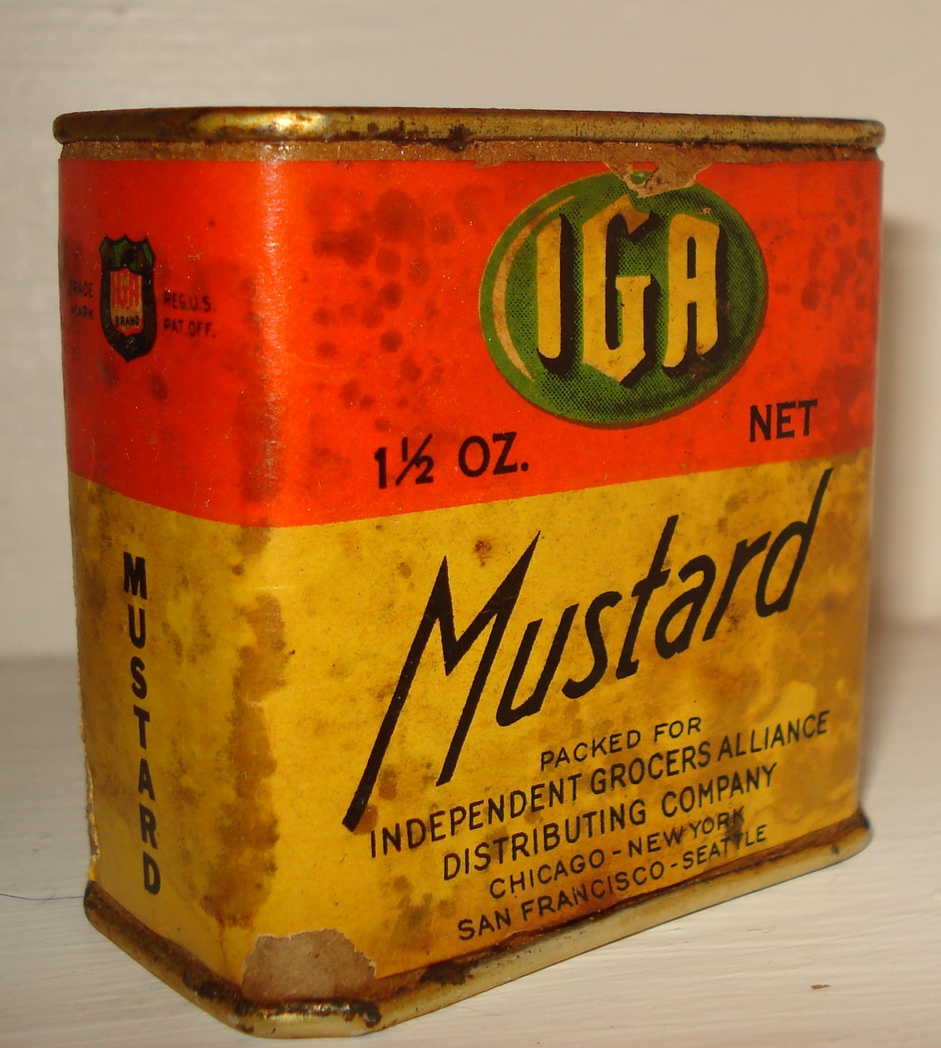This close-up photograph captures an old, vintage rectangular metal canister of IGA mustard. The canister's design features rounded edges and is wider than it is deep, presenting a nearly square face. The aging process is evident, with notable rust forming along the bottom edge and a label marred by oil stains, dirt, and discoloration. The worn label remains legible with "IGA" prominently displayed at the top on a red backdrop, accompanied by a green and white IGA logo. Below, in the lower half of the label, the text "mustard" is clearly visible, emphasizing the product contained within. The canister, originally containing one and a half ounces net, serves as a nostalgic artifact, showcasing the passage of time through its weathered appearance.